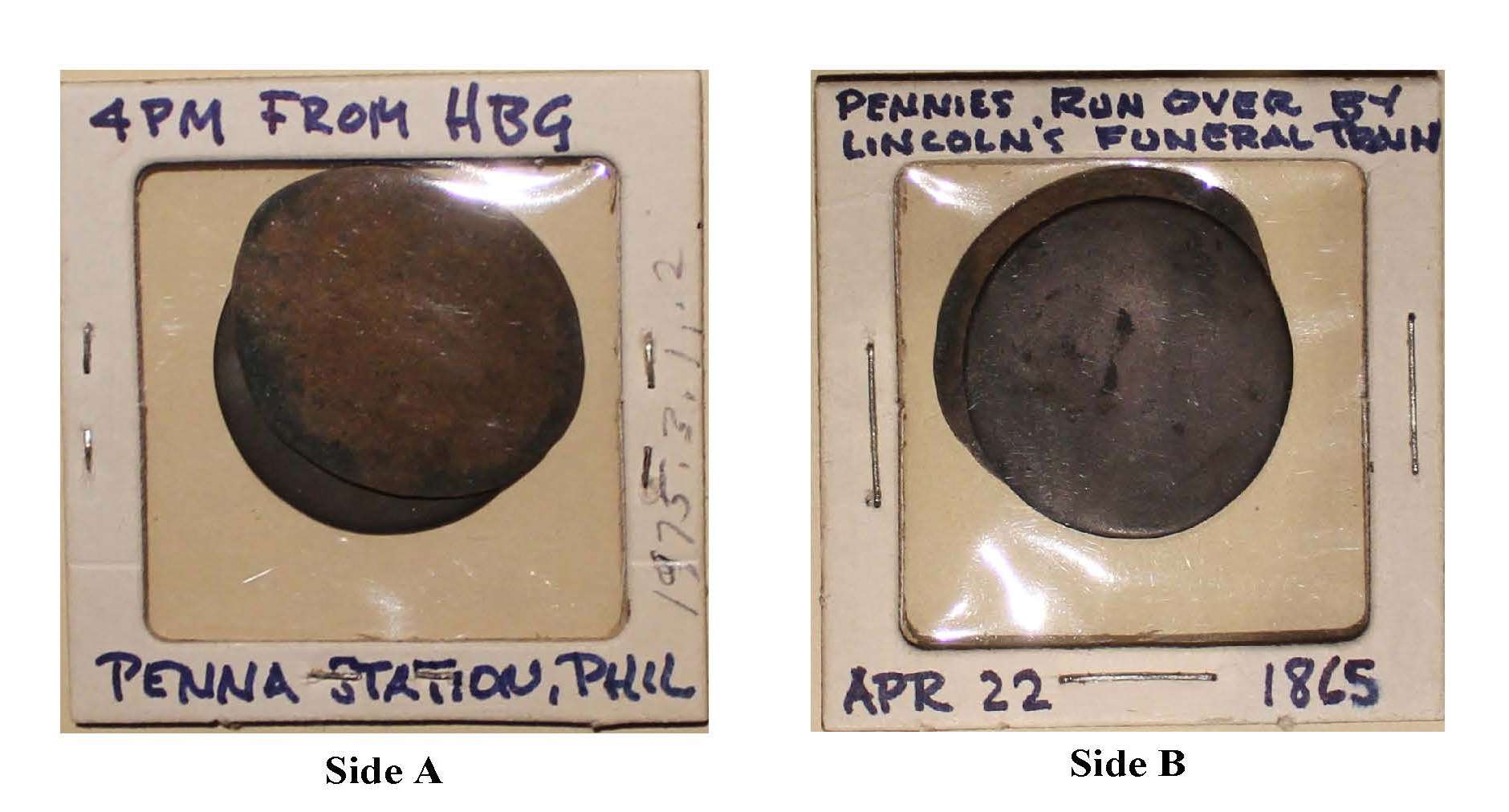This image features two antique coins preserved in paper coin sleeves with clear plastic centers. Each sleeve has a white border secured with staples.

The left sleeve has blue lettering on the top that reads "4 p.m. from HBG," with the bottom labeled "Penna Station Phil" and additional text stating "Side A." The coin within is a very old, brown, and smooth piece of metal, lacking distinctive markings, indicative of its age and wear.

The right sleeve's top label prominently states "Pennies run over by Lincoln's funeral train," and at the bottom, it says "April 22, 1865," along with the designation "Side B." Enclosed in this sleeve is a coin of a dark gray or platinum hue, resembling the moon's surface in color and texture. While there are faint, nearly indiscernible imprints on the coin, suggesting it may have had a stamped profile, the details are heavily worn away.

Both coins, although differing slightly in appearance and historical markings, are notable collectibles that appear to be cherished by the collector.